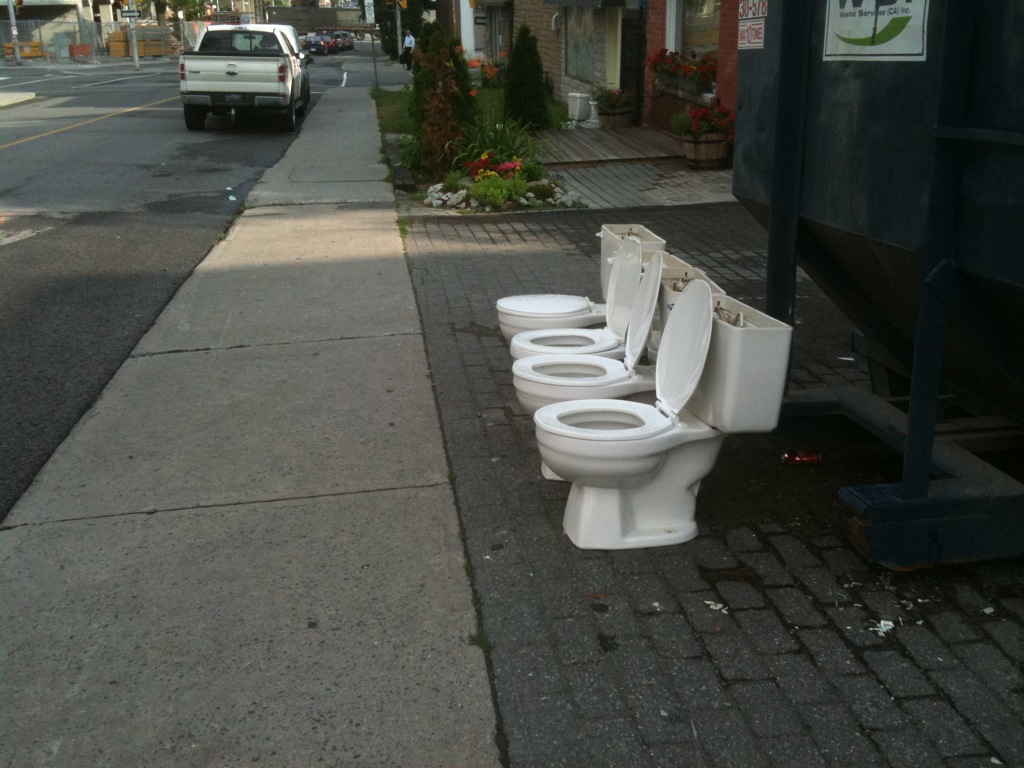The image depicts four out-of-service toilets positioned in a row on a light concrete sidewalk. All the toilets are missing their tank lids; three of the toilet seats are up, while one is down. They are situated in front of a large black dumpster, with some trash scattered around. On the left side of the image is a two-lane asphalt road where a white pickup truck, possibly with its hood up, is either parked or waiting at a corner near a stoplight. Further along the sidewalk, there's a person walking. To the right of the toilets, there's a grassy patch that includes a flower bed and some bushes. The scene appears to be in an urbanized area, possibly next to a store or a house, with a one-way street sign pointing to the right.